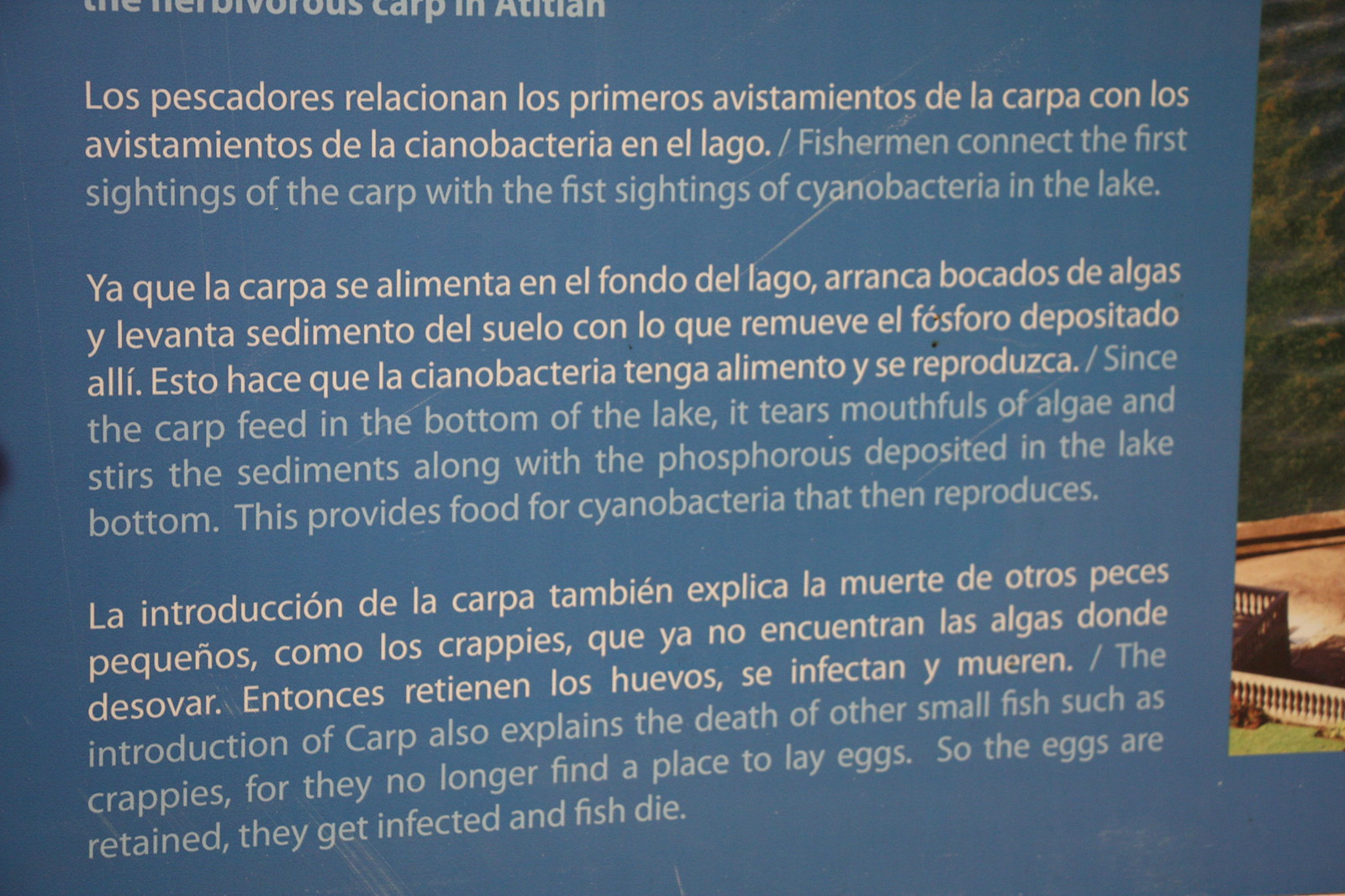This image features an outdoor bilingual sign, displayed against a blue background, containing information in both Spanish and English. The English portion of the sign title, partially obscured, suggests the topic is "Herbivorous Carp." The sign comprises three paragraphs in light blue text, detailing the ecological impact of carp in a lake. 

The first paragraph explains that fishermen have linked the initial sightings of carp with the appearance of cyanobacteria in the lake. The second paragraph describes how carp, feeding near the lake bottom, uproot and consume algae, stirring sediments and releasing phosphorus, which promotes the growth of cyanobacteria. The third paragraph discusses the adverse effects of carp introduction on smaller fish, such as crappies, who lose suitable nesting sites, resulting in retained eggs that become infected, ultimately leading to the death of these fish. 

Accompanying the text is a photograph illustrating the content. The sign highlights the complex interactions between carp and the lake ecosystem, emphasizing the detrimental impacts on water quality and native fish populations.